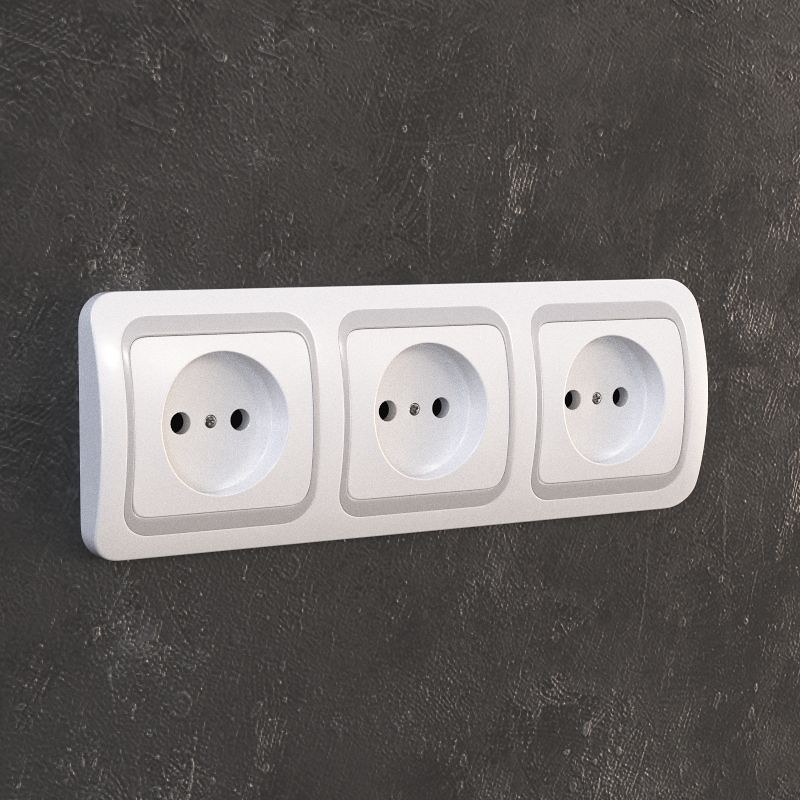The photograph displays a close-up of a black, roughly textured wall with a marbled design, featuring three white, slightly raised electrical outlets or shaving sockets lined up horizontally. Each outlet has a circular recessed area containing two circular holes, suggesting a safety feature. The design of the sockets appears to be non-American, possibly European or Asian, and might be intended for a bathroom setting. The outlets seem to be interconnected, with screws visible in the middle, securing them to the wall. The lighting in the photo is even, highlighting the subtle details of the sockets and the wall’s texture.